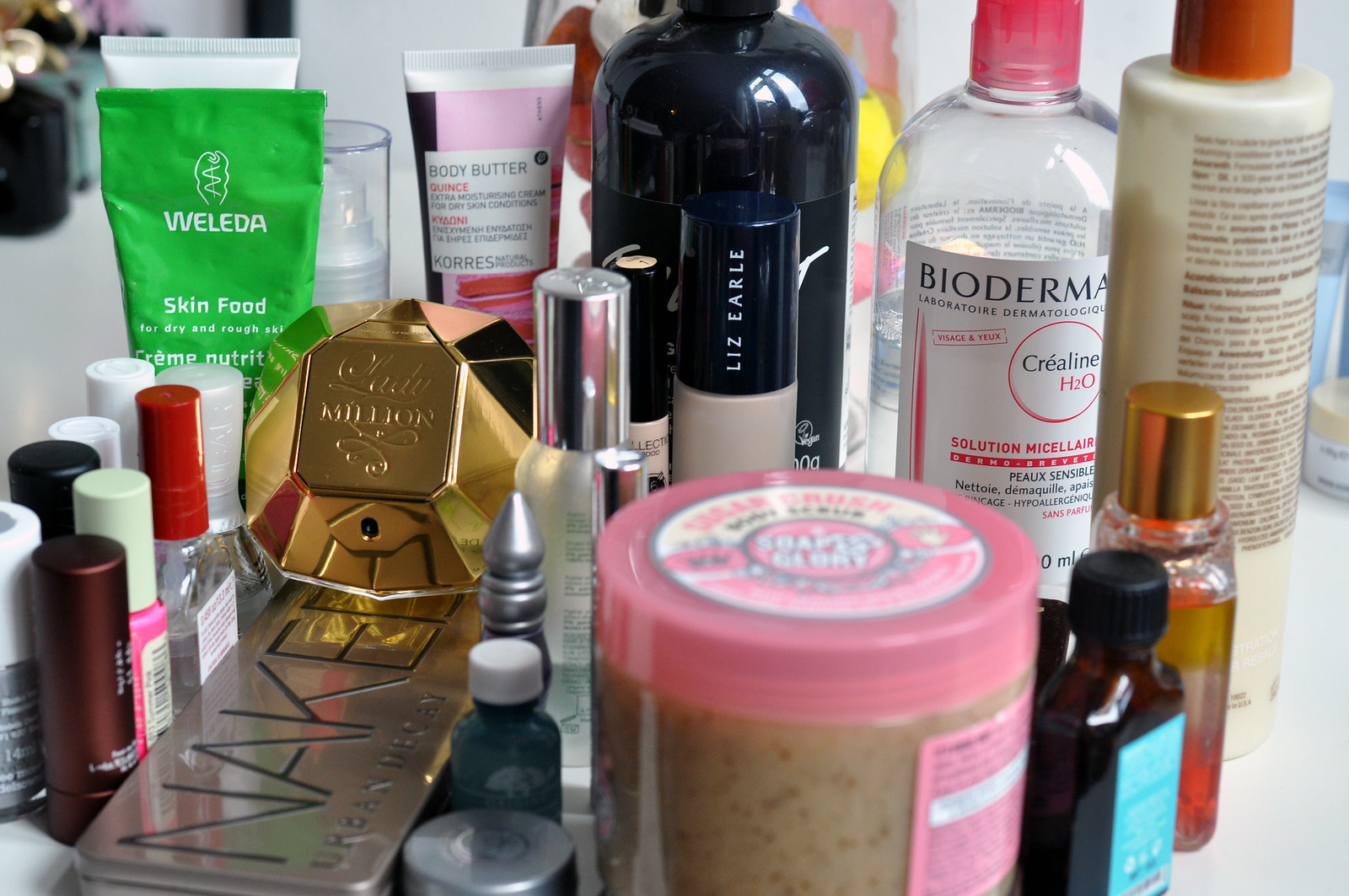The photograph is a professionally lit, horizontal color image showcasing a neatly organized collection of makeup and skincare products. The bright, clean white light highlights the various items arranged predominantly in rows.

**Back Row (from left to right):**
1. A foil squeeze tube of Weleda Skin Food in green.
2. A partially visible lotion with a pump top and a clear acrylic cap.
3. A pink and white squeeze tube labeled "Body Butter."
4. A large, dark brown or black bottle made of either glass or plastic, with an obscured label.
5. A Liz Earle product, possibly mascara or another type of makeup.
6. A clear acrylic bottle with a pink screw-on cap labeled "Bioderma Créaline H2O Solution Micellar" (micellar water).
7. Another bottle with a tan screw-on top, containing a thick, opaque white substance, likely lotion turned sideways.

**Middle Row:**
1. A gold, geodesic dome-shaped item with fancy script, possibly labeled Mildor or Kildor—the nature of the product is unclear but could be a bath bomb.
2. Various small bottles and tubes, possibly lipsticks, nail polish, or other makeup items arranged in two rows.
3. Lying flat is an item branded "Naked," potentially a case for eyeshadow or brushes.

**Front Row:**
1. A clear jar with a tan substance and brown flecks inside, likely an exfoliating product with a pink screw-on top.
2. Several small bottles typical of perfume or medicine, located on the right side of the front row.

The overall composition of the image is well-balanced, showcasing a diverse array of beauty products in a manner that suggests a well-curated personal collection.